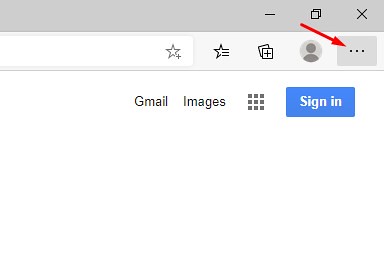In the top right corner of a Chrome browser window, the interface consists of a gray toolbar featuring the standard window control buttons: an "X" for closing, a multi-window icon for maximizing or restoring the window, and a minus sign for minimizing. Within the address bar, there's a star icon with a small plus sign, used for bookmarking the current page. Adjacent to this is another star icon accompanied by three horizontal lines, indicative of a menu or settings option.

To the right of these stars, there are two overlapping squares with a plus sign in the center, suggesting an option to open a new tab. Next to these squares, there's an outline icon resembling a head and shoulders, indicating a user profile or account options.

Further right, a gray square contains an ellipsis (dot, dot, dot), denoting a more options menu. An arrow points down from the left toward this ellipsis, drawing attention to it. 

Below this gray toolbar, the interface is white with black text. It displays "Gmail," "Images," a grid of squares representing Google Apps, and a blue "Sign in" button with white text. The rest of the image is stark white, providing no additional details or context.